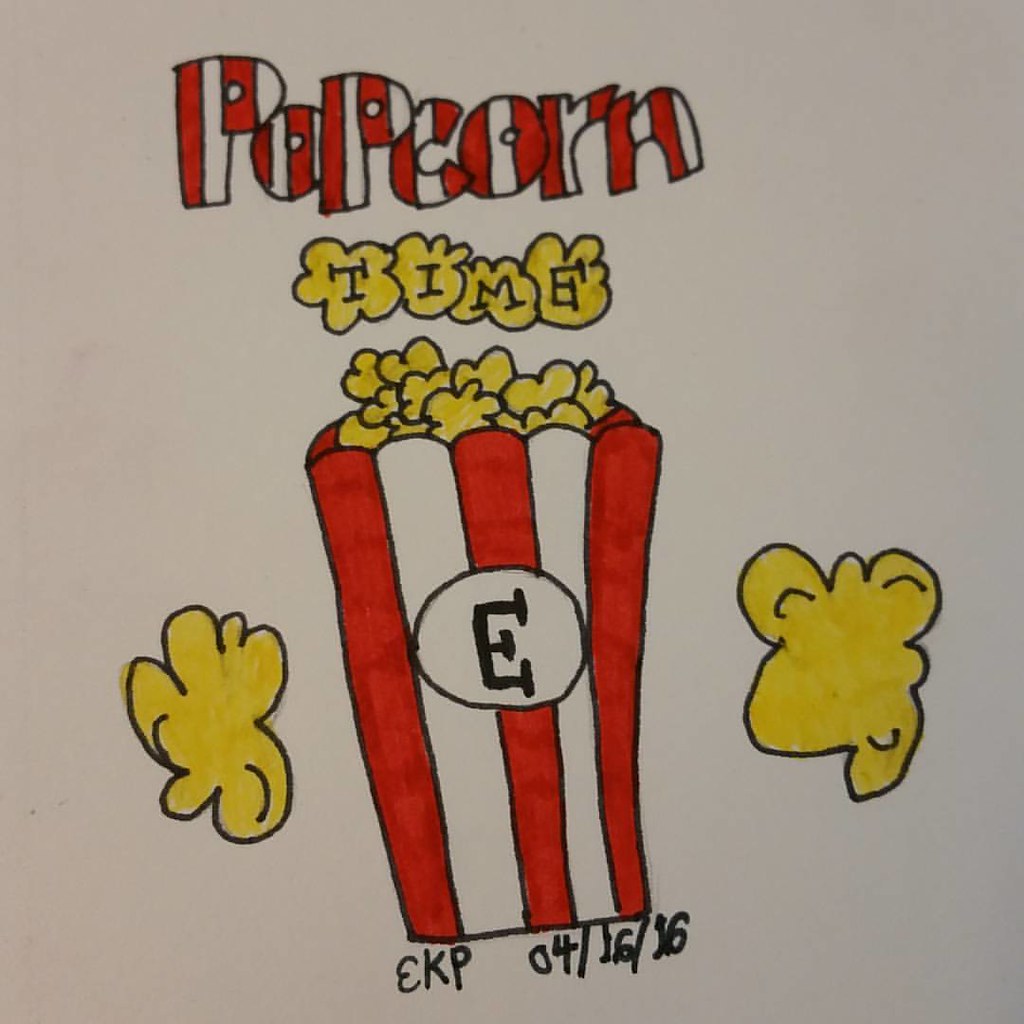This vibrant illustration, likely crafted by a young artist, depicts a classic, red and white striped popcorn box brimming with popcorn. A black letter 'E' is prominently displayed in a black circle on the front of the box, adding a personalized touch. Above the box, the word "Popcorn" is emblazoned in playful, matching red and white stripes, seamlessly blending with the box's design. Beneath "Popcorn," four plump, yellow popcorn kernels are arranged horizontally, each containing a letter that collectively spells out "Time," suggesting a playful invitation to snack time. Flanking the popcorn box on both sides, additional large golden kernels add to the illustration's whimsical feel. Below the popcorn box, the text "EKP 04-16-16" is written, potentially indicating the artist's signature and the date of creation. The entire image exudes a cheerful, nostalgic vibe, reminiscent of a fun day at the movies.